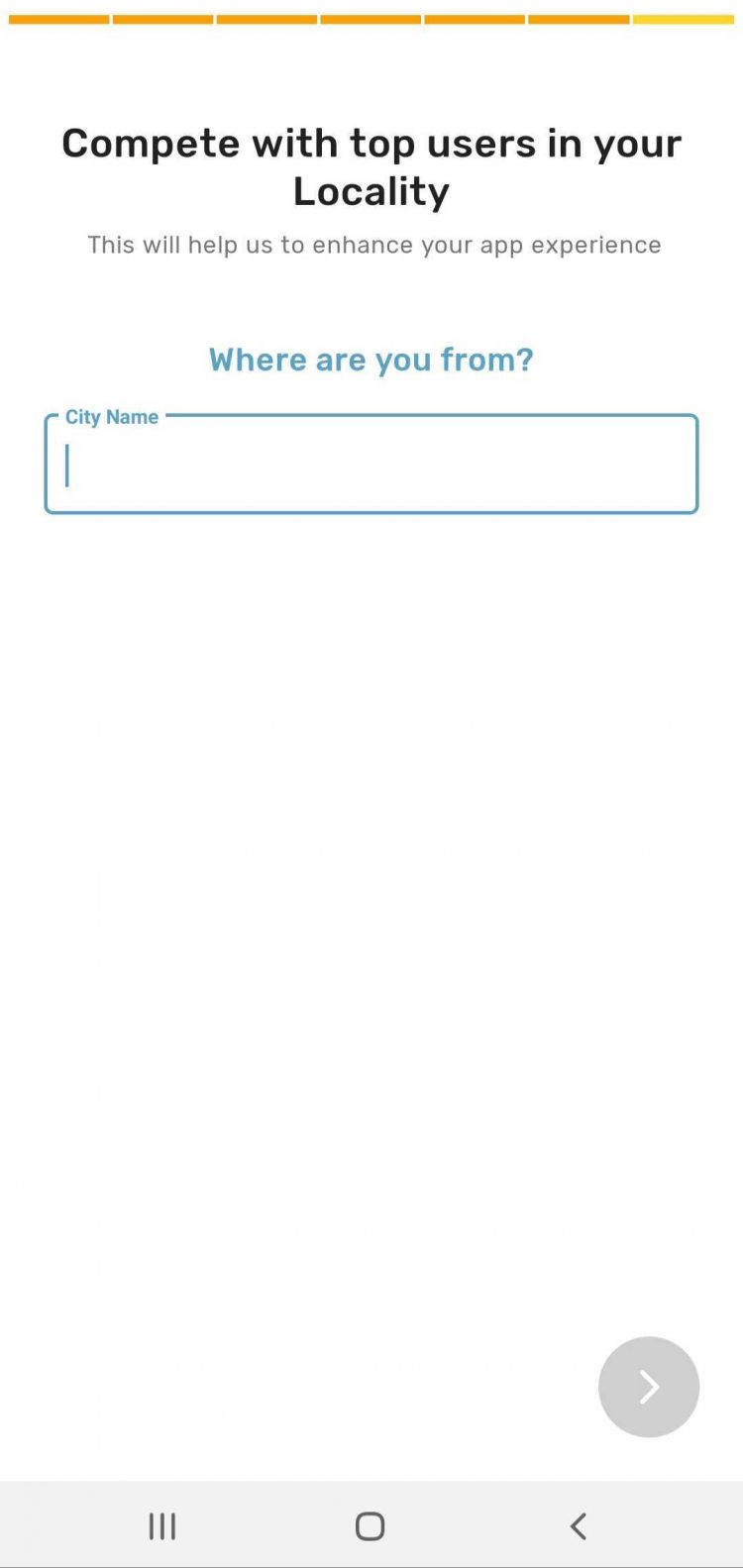The image features a UI layout showcasing a series of text prompts and input fields in a clean, structured format. At the top, a broken, gradient yellow line transitions from a darker shade on the left to a lighter shade on the right. Approximately two to three inches below this line, the text "Compete with top users in your locality" is prominently displayed in bold black. Below this statement, a lighter gray text reads, "This will help us to enhance your app experience," providing additional context for users.

Further down, about three inches below the initial text, a prompt in blue text asks, "Where are you from?" Directly underneath this question, there is a rectangular input field to enter information. At the top left of this field, small blue text reads "City name," next to which is a small vertical line for separation.

About six inches down from this point, the layout includes a right-facing arrow enclosed within a light gray circle. Positioned to the left of this icon are three small vertical lines, a square in the center, and an arrow pointing from left to right. The entire section is underlined by a light gray line, providing a clean division from the rest of the layout.